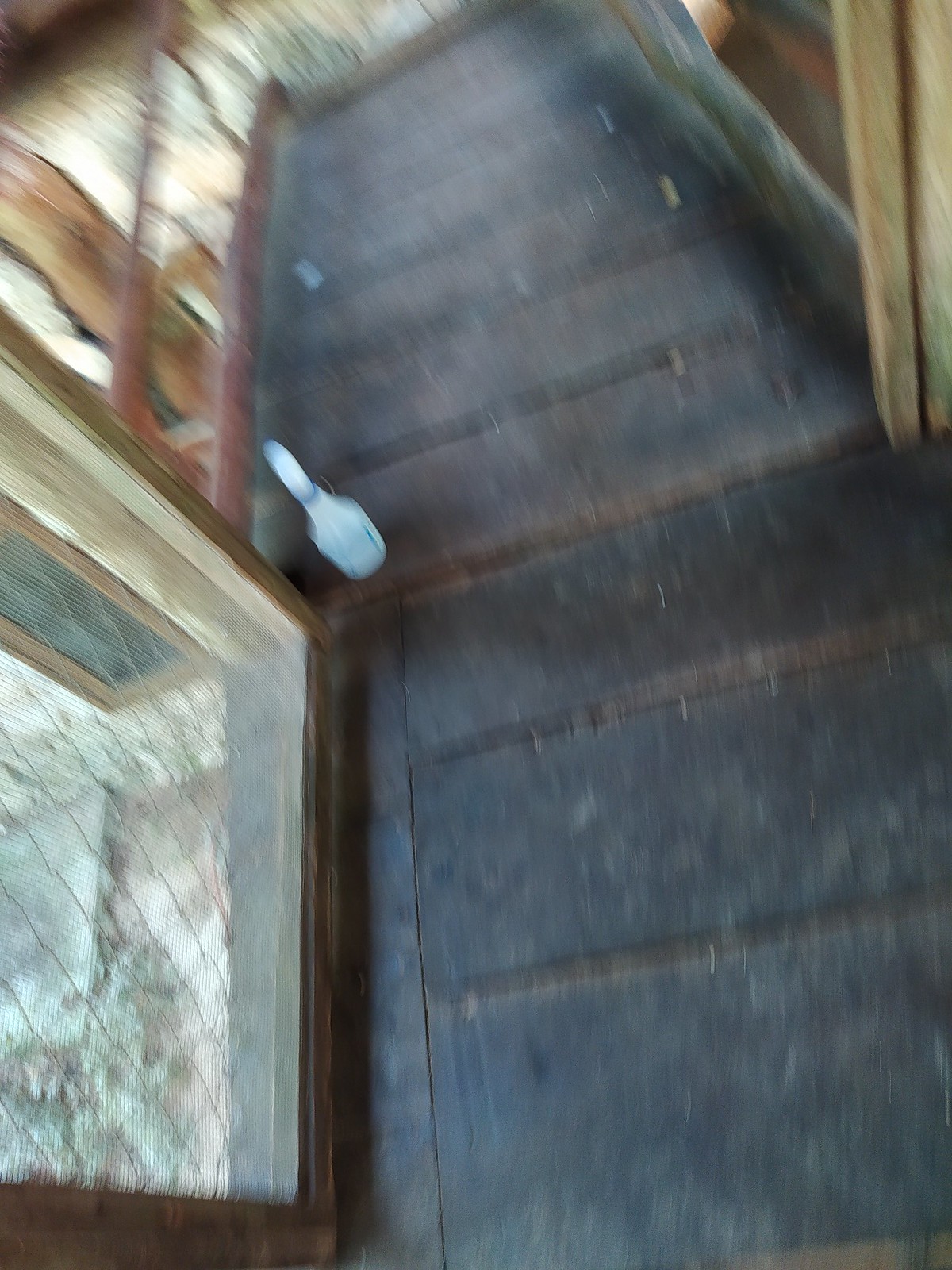The photograph captures a slightly angled, downward view of a dark gray or black wooden walkway with deep grooves, giving it a striped appearance. The daylight streams through to the left side of the image, illuminating a section of the scene with a diffused glow. On the left side of the walkway, a wooden structure resembling a door frame extends upward, and within it, we can observe a chain-link fence. This combination of elements suggests we might be inside or near an enclosed area potentially meant for animals, such as a viewing area or a part of a chicken coop.

Moving towards the center of the image, we spot a small spray bottle placed on the floor. Adjacent to the walkway, a blurred red metal railing stretches into the background, indicating the presence of a raised gantry or pathway. The image also features several wooden posts—one vertically oriented on the right side—contributing to the framing of the scene. Although the background fades into a blur, a distinct patch of white light is visible beyond the railings on the left, adding contrast and depth to the composition.